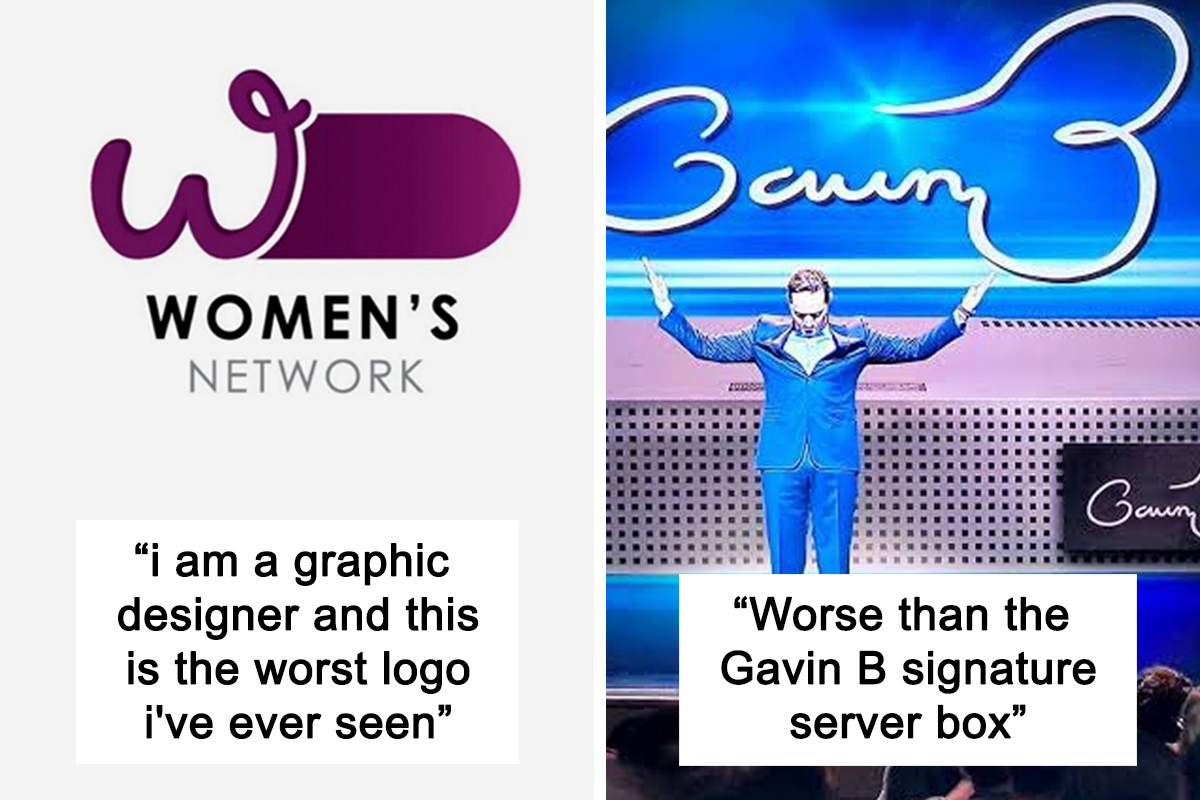The composite image consists of two sections placed side by side. On the left, a simplistic, white-background image features a large, purple "W" logo with the text "Women's Network" written beneath it in black, lowercase letters. Below this, a quote states, "I am a graphic designer and this is the worst logo I have ever seen." The right section showcases a man in a blue suit standing on a stage with his arms raised. Above him, there's unrecognizable, cursive-like text, making only the letter "3" discernible. Near this man's knees, another quote reads, "Worse than the Gavin B signature server box." In the background, some members of an audience are partially visible, suggesting he is addressing a crowd.